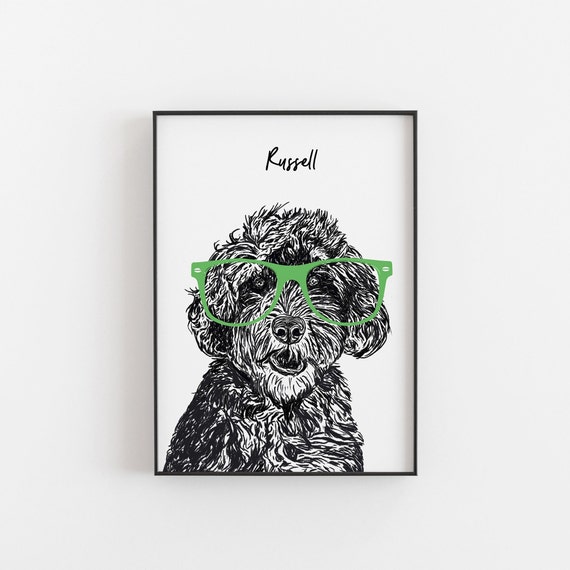This is a detailed image of a framed artwork depicting a dog, mounted on a white wall. The artwork features a thin black metal frame surrounding a white background. The central focus is a sketched, black and white drawing of a dog that resembles a poodle mix, possibly a Labradoodle, due to its distinctive curly and shaggy fur. The fur around the dog's face is particularly wild and tousled, casting shadows around its eyes. The dog’s expressive face is accentuated with oversized green glasses that sit humorously large on its face, adding a splash of color to the monochromatic sketch. These glasses are so big that they extend beyond the sides of the dog’s face, making its eyes appear black from behind the lenses. The dog is facing forward with its mouth slightly open, giving the impression that it's smiling straight at the viewer. Above the dog's head, in black cursive font, is the name "Russell," suggesting that this is the dog's name. The entire image is a close-up, showing the dog's upper body and face in fine detail.